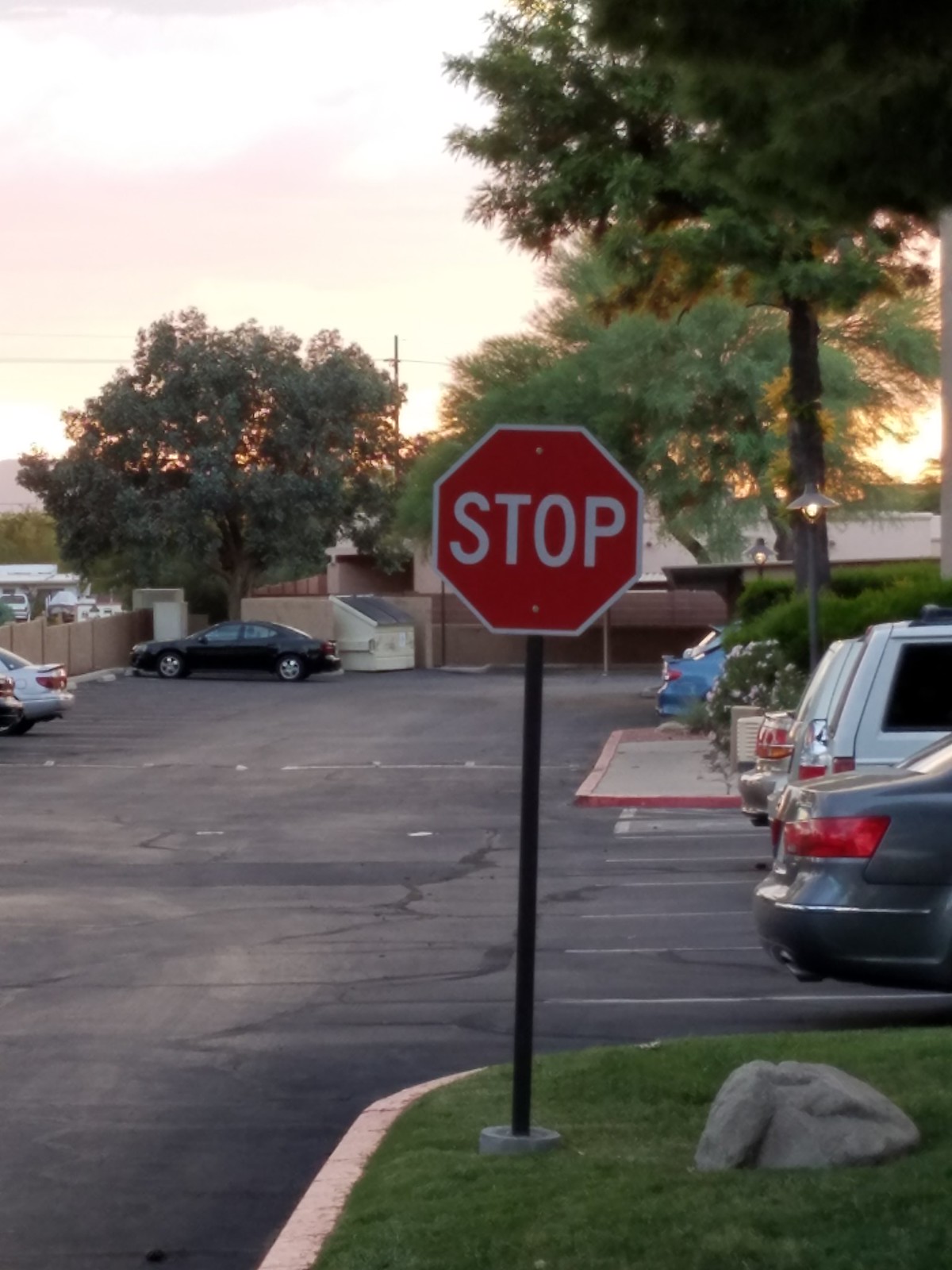In this vertical rectangular photograph, we see a parking lot at what appears to be the setting or rising sun, casting a bright light across the scene. Dominating the center of the image is a red stop sign with white lettering, mounted on a black pole cemented into a block on a grassy median. Flanking the stop sign on both sides, cars are parked orderly within white-lined parking spaces, with the right section showing the rear ends of a gray sedan with red taillights, a taller white SUV or minivan, and a distant blue car. The left side features cars facing inward, including a white vehicle and a black one further back. Large, green trees line the background with some visible on the upper right corner of the image, while a brown fence is positioned in front of a black car. Additionally, a grey garbage can and a tan dumpster with a black plastic lid can be seen behind the vehicles. The parking lot, bordered by a black asphalt driveway, appears to be adjacent to a business building partially visible in the background. Overall, the photograph captures a typical parking lot scene with detailed elements such as the greenery, vehicles, and structural features.